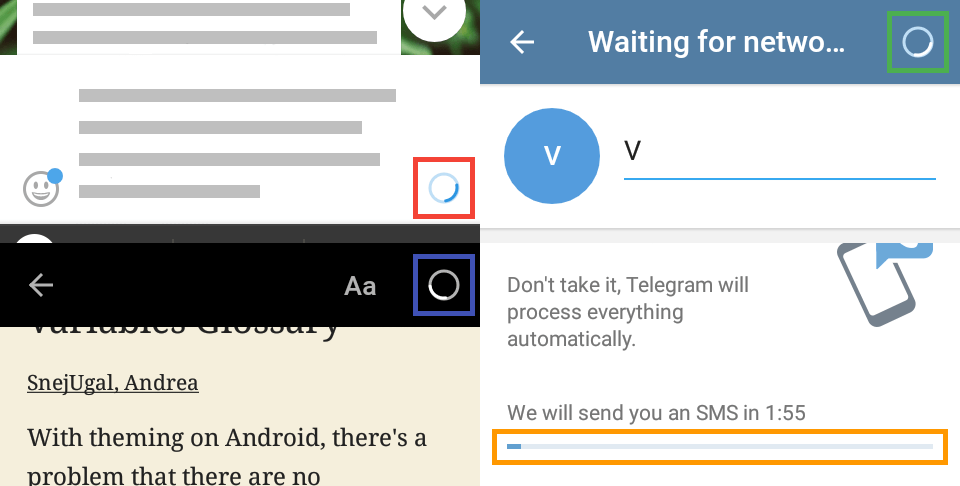This is a detailed caption for the provided image of side-by-side screenshots:

---

**Detailed Caption:**

The image consists of two side-by-side screenshots of a website, each with distinctive features. 

**Left Screenshot (Vertical Rectangle):**
- **Top Half**: 
  - Background: Predominantly white.
  - Top Left Corner: Contains a small section with a black background featuring a green leaf and a vertical rectangle image.
  - Paragraph: A single paragraph with text on a gray background, partially obscured by horizontal gray stripes, located next to the small rectangle image.
- **Middle Section**: 
  - Image: To the left, there is an image of a gray smiley face with a blue dot at the top right.
  - Text: To the right of the smiley face, another paragraph is visible but has been obscured (or canceled out) with three long horizontal blue-gray stripes and a fourth stripe that is three-quarters the length of the others.
- **Lower Section**: 
  - Black Horizontal Rectangle: 
    - Left Side: Features a left-facing white arrow.
    - Center: Displays a gray capital 'A' and a lowercase 'a'.
    - Right Side: Contains a blue outlined box filled with black and a white circle inside.
  - Text: Beneath the black rectangle, there is some cut-off text. The visible part, to the left, reads "Snedugal Andrea" in underlined black letters. Below this, more text appears, stating, "with theming on Android there's a problem that there are no," followed by a cut-off point. 

**Right Screenshot (Horizontal Rectangle):**
- **Top Section**: 
  - Background: A horizontal blue rectangle at the top.
  - Left Side: Includes a left-facing white arrow.
  - Center: Contains the text "waiting for N-A-T-W-O" followed by three dots.
  - Right Side: Features a green outlined box filled with blue, containing a white circle.
- **Middle Section**: 
  - Icon: A blue circle with a white 'V' inside.
  - Text: To the right, a black 'V' with an underline trailing off to the right across the page in blue.
- **Lower Section**: 
  - White Horizontal Rectangle:
    - Top Left: Contains the text "don't take it, Telegram will process everything automatically" in gray.
    - Middle: States, "We will send you an SMS in 1 minute 55 seconds."
  - Orange Outlined Rectangle: 
    - Contains a progress bar filled approximately five percent.
  - Right Side of Page:
    - Shows an outlined, left-tilted cell phone in dark blue or dark gray. The screen area is white, with part of a blue message button visible and cut off at the top right.

---

Each section of the screenshots provides visual and textual elements indicative of the website's interactive and messaging features while displaying partially obscured information.